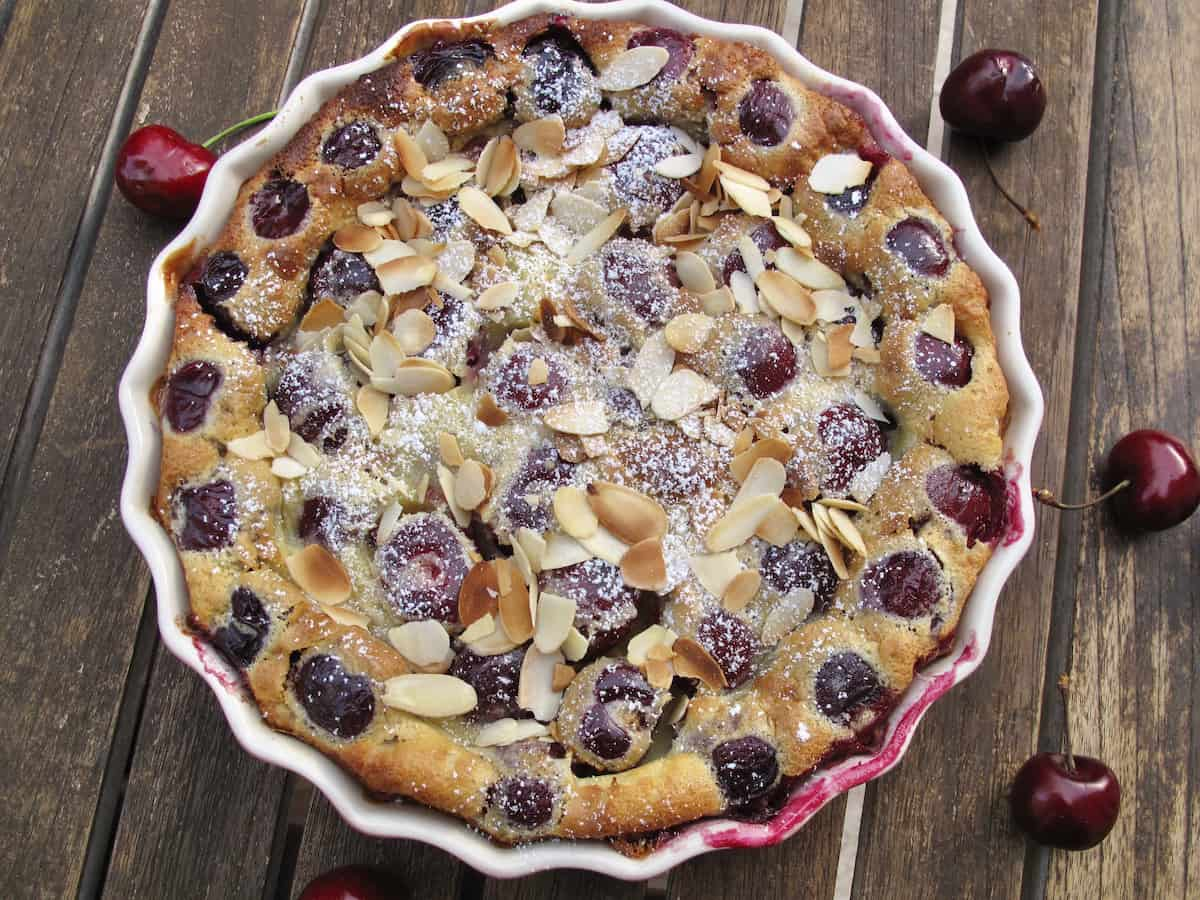This top-down photograph captures a cherry pie placed in the center of a white, scalloped-edged pie plate on a dark walnut wooden table with vertical planks. The pie features a golden-brown crust, dusted with powdered sugar, and is adorned with dark red cherries both inside and on the crust, where thin slices of almonds are scattered. Surrounding the plate, cherries with green stems are positioned at various spots across the table—three on the right-hand side, one on the top-left corner, and a few others strategically scattered, enhancing the vibrant and appetizing presentation of the pie.